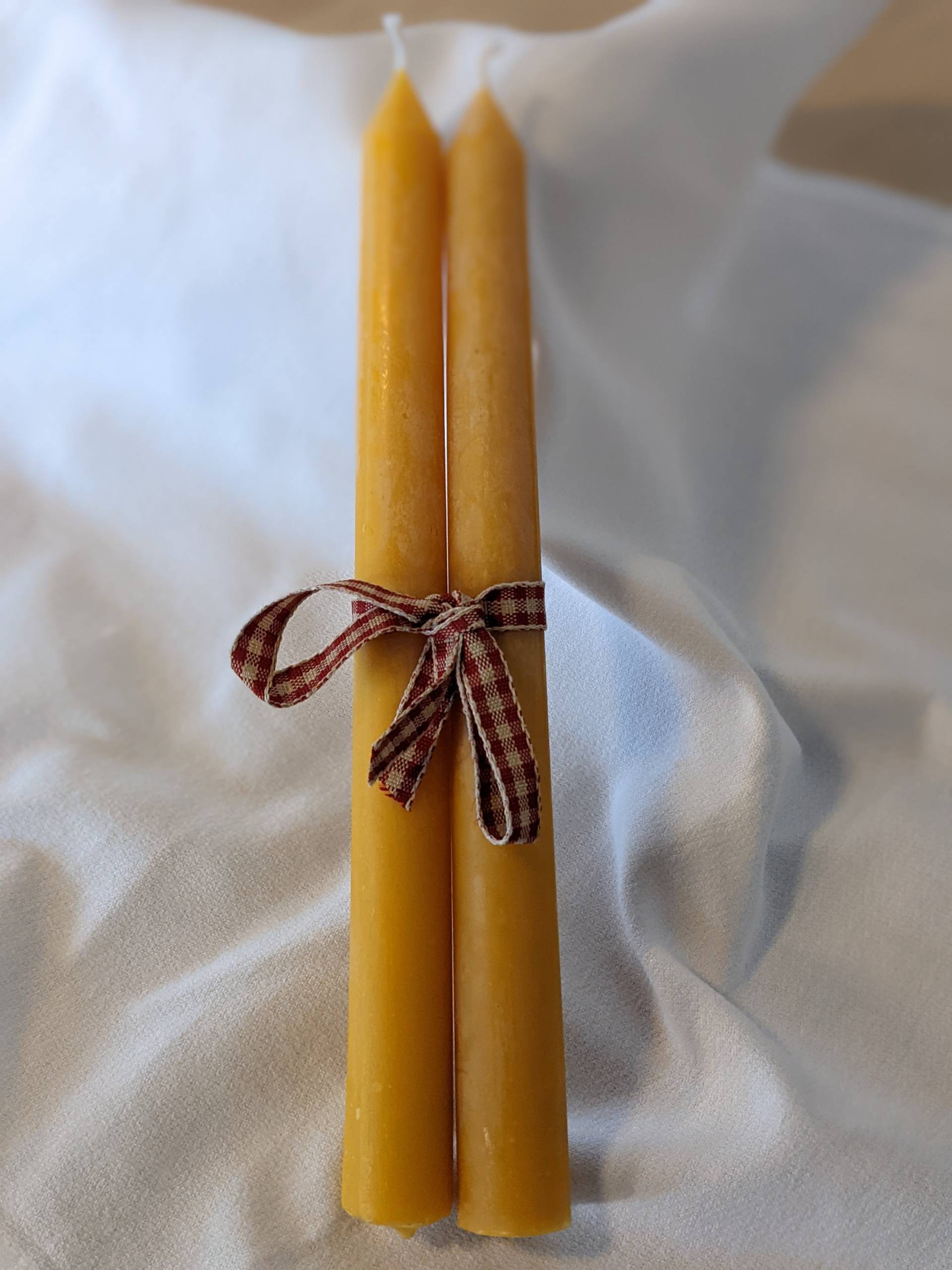The image captures two long, amber-colored candles with white cloth wicks, reminiscent of those used in old-fashioned candelabras. These candles are approximately 12 inches in length and lie side by side. They are elegantly bound together with a checkered ribbon, featuring a maroon and tan pattern that evokes a vintage or picnic cloth design. The ribbon is tied into a neat bow, adding a touch of rustic charm. Both candles are positioned on an off-white cloth, which is slightly crumpled and creates visible ripples. The background of the image includes what appears to be a wooden surface or table, partially visible in the upper portion of the frame. The overall scene is softly lit, casting gentle shadows that accentuate the texture of the crumpled cloth.